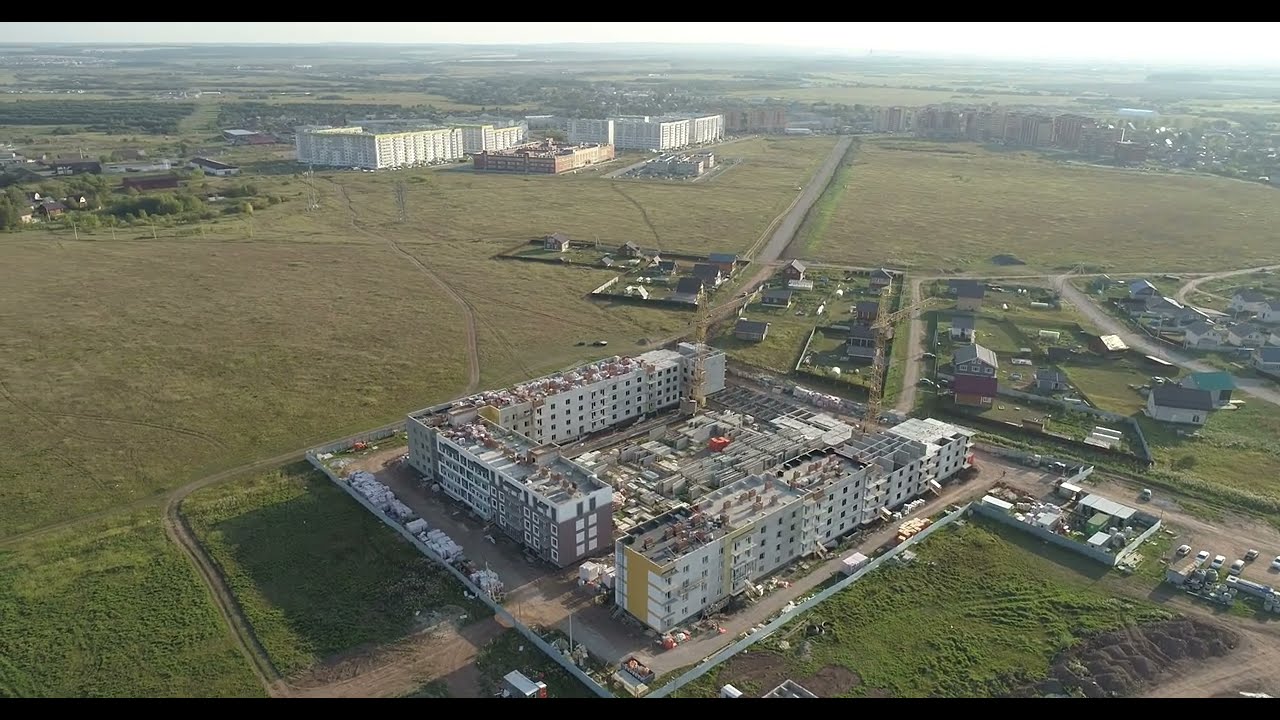This overhead view captures a rural town or a sparsely populated city area showcasing a mix of buildings at different construction stages. At the forefront, a multi-unit residential complex is under construction, characterized by structures reaching the 4th floor, flanked by cranes suggesting ongoing development. These buildings are composed of white facades with grid-shaped windows, alongside brown two-level structures. In between these buildings, the ground is occupied by construction equipment and ladders rather than open green spaces or parking lots. Surrounding the construction site are smaller, single-family farming homes, typical of a rural setting. The photo also reveals a road that stretches into the horizon, leading to a city skyline miles away, with additional buildings dispersed in the background. The landscape is punctuated by open fields and greenery, providing a stark contrast to the varying colors of the buildings, predominantly white, green, brown, and hints of blue. Overall, this image depicts a developing town with residential and possibly educational or working centers, set against a bucolic backdrop.